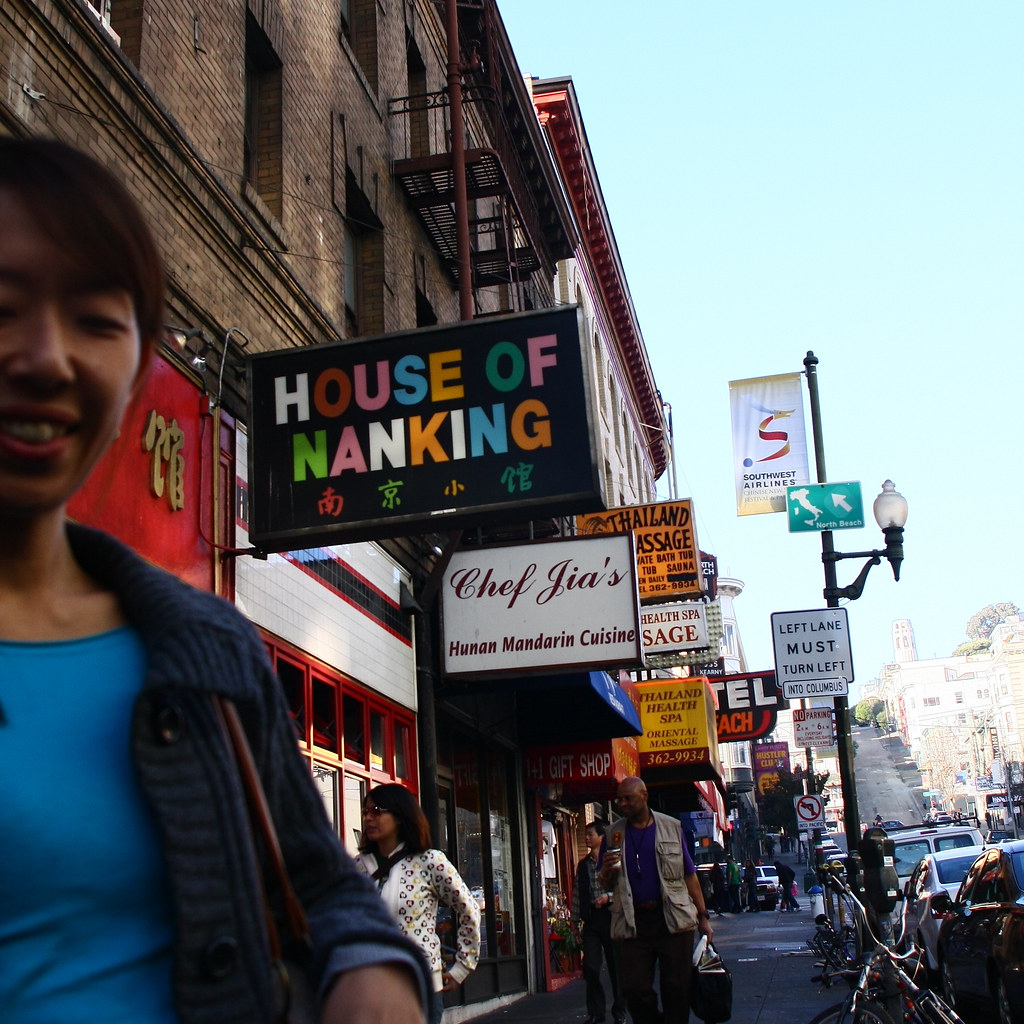The image captures a vibrant street scene, likely set in Thailand, evidenced by the "Thailand Massage" sign. The scene is populated with a variety of colorful signs, including "House of Nanking" in multi-colored letters with Chinese symbols, and "Chef Jia's Hunan Mandarin Cuisine." The street is bustling with activity: cars are parked alongside, and several pedestrians are visible, including a tall man in a beige sleeveless jacket and a bag, and a woman in a spotted white blouse with a scarf. In the foreground, on the left, a woman with an open blue shirt and buttoned sweater appears to be taking a selfie, smiling down at the camera. The setting is sunlit, with a clear blue sky overhead. The street itself slopes upward, with a lamppost and various parking signs visible. There are bikes parked on the sidewalk and large brick and stone buildings stretching into the distance, lending a sense of depth and indicating a potentially bustling neighborhood. The abundant signage and diverse crowd suggest a lively, multicultural locale.